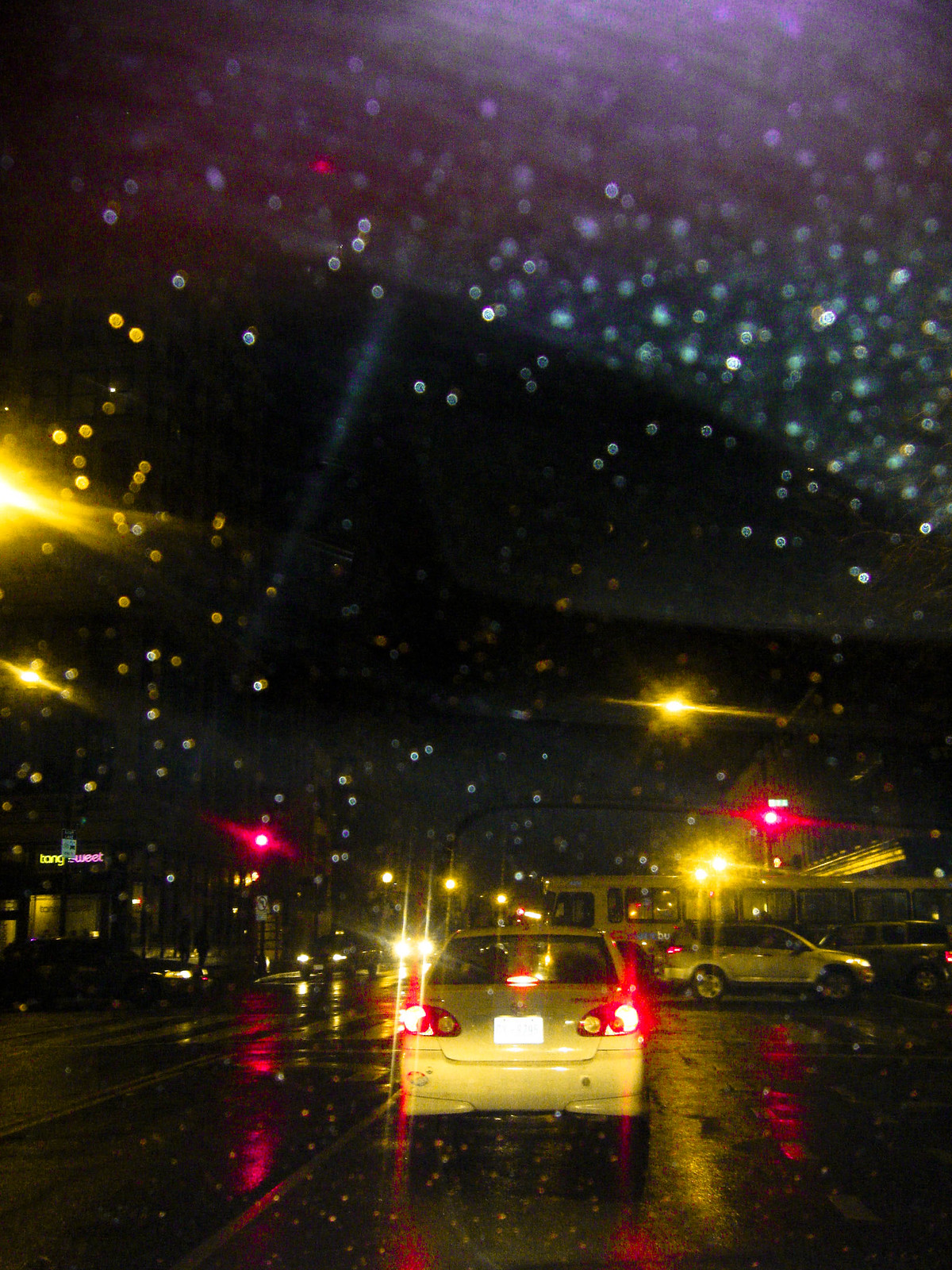In this nighttime scene captured from inside a car, the rain-spattered windshield reveals water droplets and smears from the windshield wipers. The darkness envelops the surroundings, but a cluster of streetlights provides illumination. The yellow and red glow from traffic lights punctuate the scene, casting reflections on the wet asphalt. 

Central to the image is a small white car, its red brake lights casting a vivid contrast against the darkness. Ahead of this vehicle, other cars are visible, some moving towards the camera while others traverse the intersection perpendicularly. A large bus can be seen crossing through the traffic light, adding to the busy nighttime traffic scene. 

To the left side of the frame, a business named "Tang Sweet" can be discerned, its sign barely visible due to the low light conditions. The overall ambiance of the photo reflects a quintessential rainy night in the city, filled with the hustle and bustle of vehicles navigating through glistening streets.